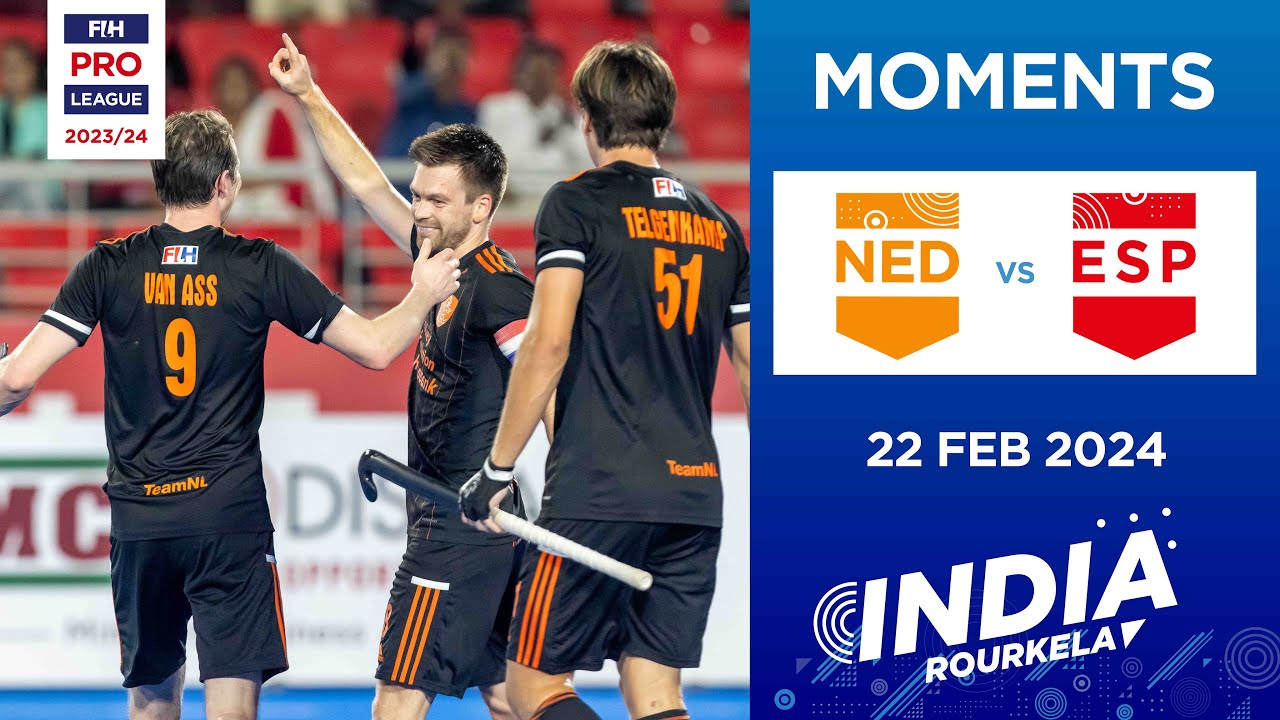This image is an advertisement for the FIH Pro League 2023-24 featuring a memorable moment from the NED vs. ESP match held on February 22, 2024, in Rourkela, India. The left two-thirds of the picture captures a celebratory scene of three athletes, all dressed in field hockey uniforms, basking in their triumph. One player, prominently positioned in the middle, points upwards with a "number one" gesture, suggesting they have scored a significant goal or won the match. His two teammates, with their backs to the camera, flank him in spirited support. The background of this section shows blurred-out sports fans, enhancing the excitement of the scene. On the right one-third, against a blue backdrop, the text details the event information, including "Moments," "NED vs. ESP," and "22 February 2024," with "India, Rourkela" clearly emphasizing the location and date of this remarkable sporting moment.